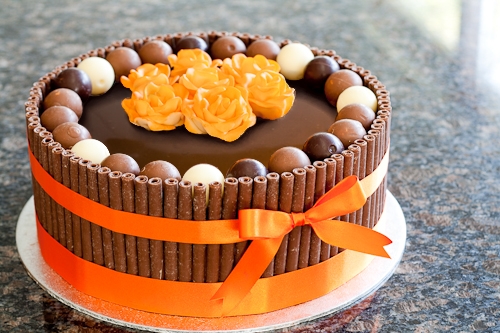This image is a color photograph of a meticulously decorated chocolate cake, likely reminiscent of a high-end bakery creation or an advertisement for an online confectionery. Enveloped around the cake is a striking presentation of what seems to be chocolate shavings or wafer-like tubular cookies, giving the appearance of a fence that extends above the cake's surface. These structures are secured by two satiny orange ribbons—one at the base and another about two-thirds up the cake, each tied in neat bows accentuating the decorative elegance.

The top surface of the cake is cloaked in a smooth layer of dark chocolate fondant, bordered inside the chocolate fence by a variety of gumball-sized chocolate balls, possibly bonbons or malt balls. These come in a harmonious mix of white, light brown, and dark brown hues, adding to the visual and textural intrigue.

Crowning the cake is a splendid arrangement of seven frosting roses—six forming a hexagonal pattern with one central rose—all in a vibrant orange that matches the ribbons. This intricate display rests on a reflective silvery platter positioned on a countertop which appears to be made of granite with diverse shades of blue, orange, yellow, and beige, offering a sophisticated backdrop to the sumptuous cake.